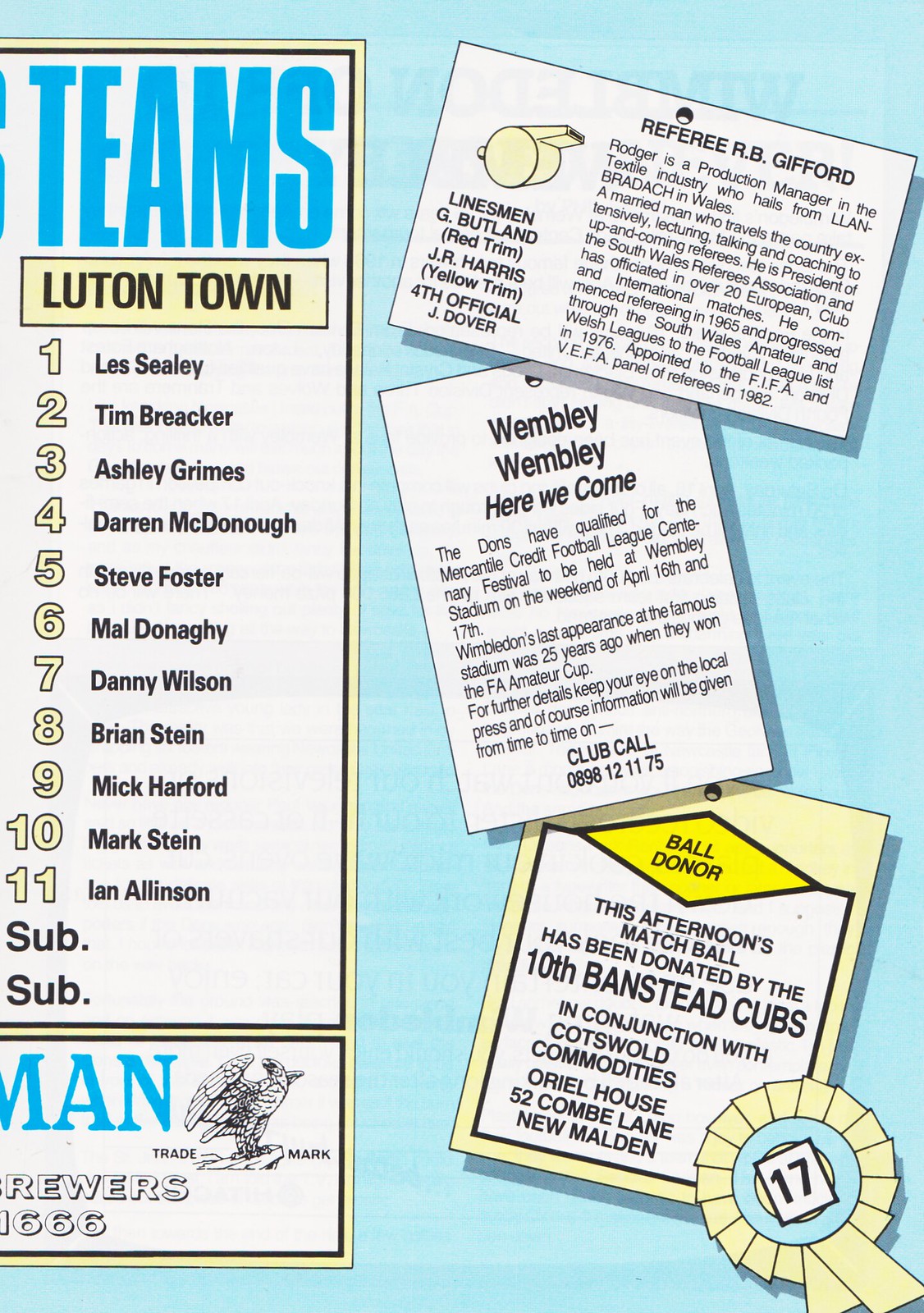This image appears to be a digitally remastered old-school sports advertisement, prominently featuring a team lineup and various informational elements. The left side lists the lineup for "Teams: Luton Town," including eleven players: Les Seeley, Tim Breacker, Ashley Grimes, Darren McDonough, Steve Foster, Mal Donaghy, Danny Wilson, Brian Stein, Mick Harford, Mark Stein, and Ian Allenson. The right side of the image contains additional details, such as "Wembley, Wembley, here we come," and mentions the ball donor: "This afternoon's match ball has been donated by the 10th Banstead Cubs in conjunction with Cotswold Commodities, Oriole House, 52 Combe Lane, New Malden." A ribbon with the number '17' and a small, somewhat elusive text hinting at a referee named RB Gifford, adds further vintage touches. At the bottom left, there is an eagle emblem with "trademark" on each side, reinforcing the old-fashioned style of the advertisement. The image utilizes a palette of light blue, blue, white, yellow, black, and grey, and is graphically designed to resemble an advertisement or informational poster from the 1950s.